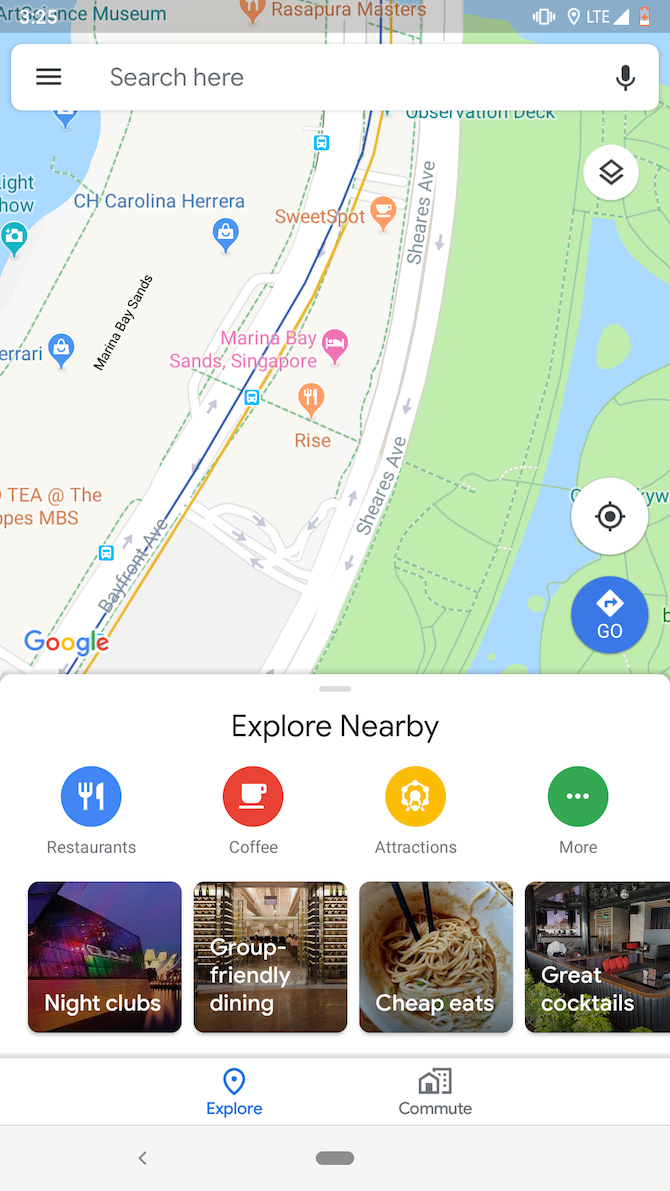This is a rectangular image oriented vertically, depicting a map displayed on a smartphone screen. At the top of the screen, a semi-transparent gray status bar displays the time as 3:25 on the left side, along with several icons on the right: a vibrate icon, LTE service indicator with full signal bars, and a red battery icon indicating a low charge. Below the status bar is a search bar featuring a hamburger menu icon on the left, placeholder text reading "Search here" in the center, and a microphone icon on the right.

The map occupies the main portion of the screen, showing an area with bodies of water located in the upper left and right-hand sections. Various roads traverse the map. In the lower section of the map, there are four circular icons each representing different categories of locations: a blue icon with a knife and fork for restaurants, a red icon with a coffee cup for coffee shops, an orange icon with a Ferris wheel for attractions, and a green icon with three horizontal dots suggesting more options or miscellaneous categories.